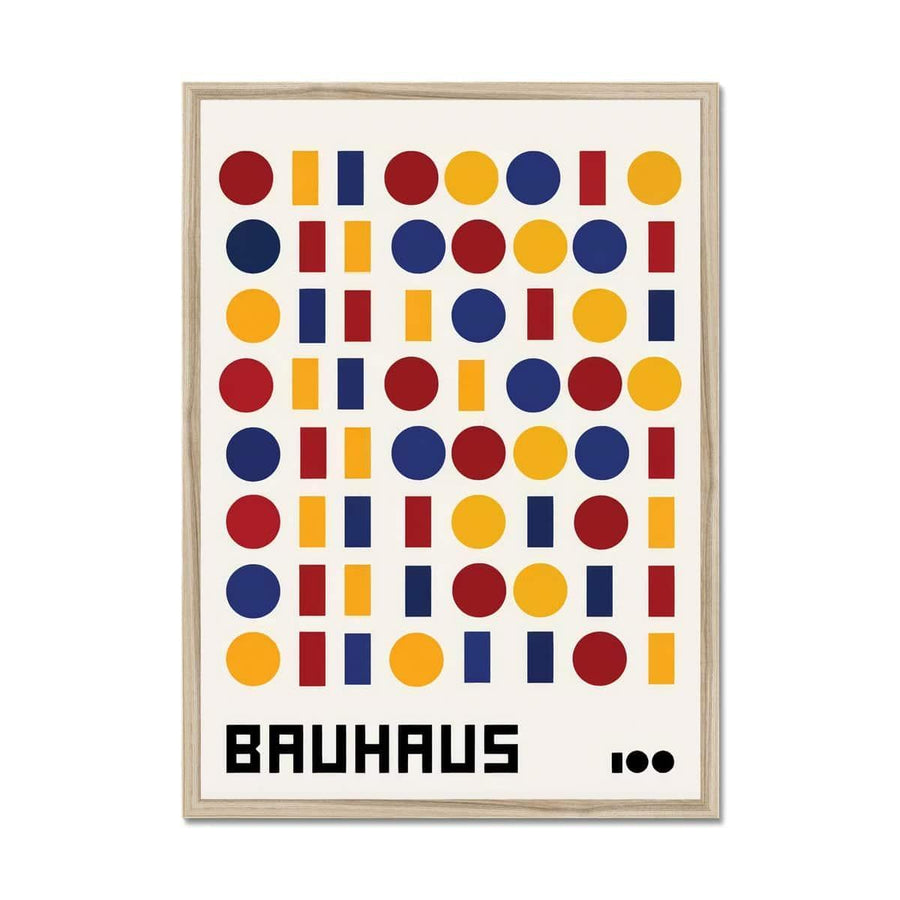This is a large white-framed poster with a bright white background, featuring an arrangement of colorful shapes such as circles and rectangles. The shapes, colored in red, yellow, and blue, are distributed across the entire poster in varying sequences. Sometimes, they appear in rows of circles or rectangles, and other times in mixed patterns. In the bottom left corner, the word "Bauhaus" is written in black letters, while the bottom right corner contains a small rectangle and two small circles in black. The frame is a whitewashed wood color, adding a subtle texture that complements the vibrant simplicity of the poster's design.